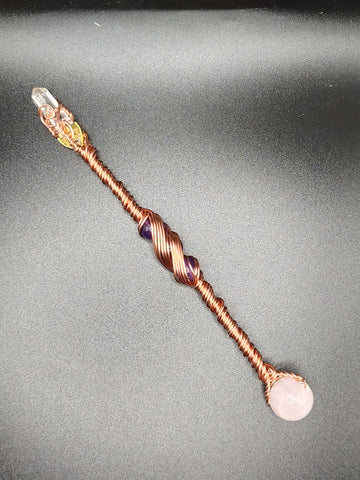The photograph captures a vertically oriented, bar-like object made of intricately coiled copper wire, resembling a miniature, fantastical staff or wizard's wand. The object stretches from the top left to the bottom right of the image. At the upper left end, a slender quartz crystal is set into the copper wire, adding a mystical touch. The center of the staff features a thicker winding adorned with small, purple beads, giving the impression of a handle. At the bottom right end, the wire forms a delicate filigree design around a spherical bead, which appears off-white with a possible pinkish hue. The entire object is set against a light gray background that transitions to medium gray on the right side and fades to black towards the top edge of the image. The composition of the photograph, a vertical rectangle, enhances the slender and elongated nature of the copper-wire creation.